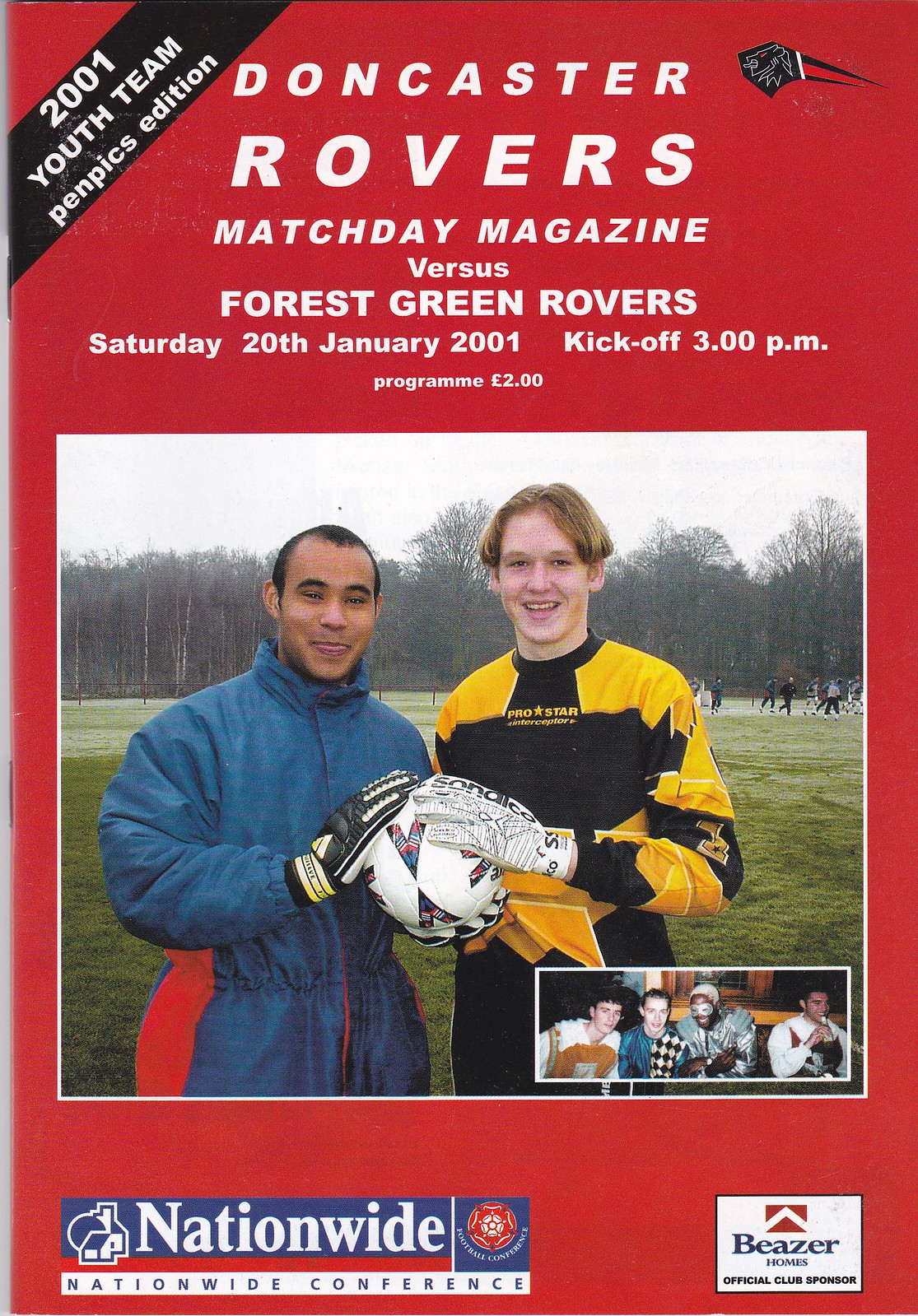The front cover of this Match Day magazine for a football game features a vibrant red background. In the top left corner, the text reads "2001 Youth Team Pen Picks Edition," and at the top center, it states "Doncaster Rovers Match Day Magazine versus Forest Green Rovers," with details "Saturday 20th, January 2001, Kickoff, 3 p.m., Program, £2" in white font. The center of the page showcases an image of two soccer players, likely goalies due to their attire. One is in a blue outfit with black gloves and holds a soccer ball, while the other wears a black uniform with yellow accents and white gloves, also holding a ball. They are standing on a grassy field with trees and additional players in the background. In the bottom right corner of the image is a smaller photo featuring four people smiling and enjoying themselves. The bottom of the cover lists "Nationwide Conference" and mentions "Beezer Homes, official club sponsor."